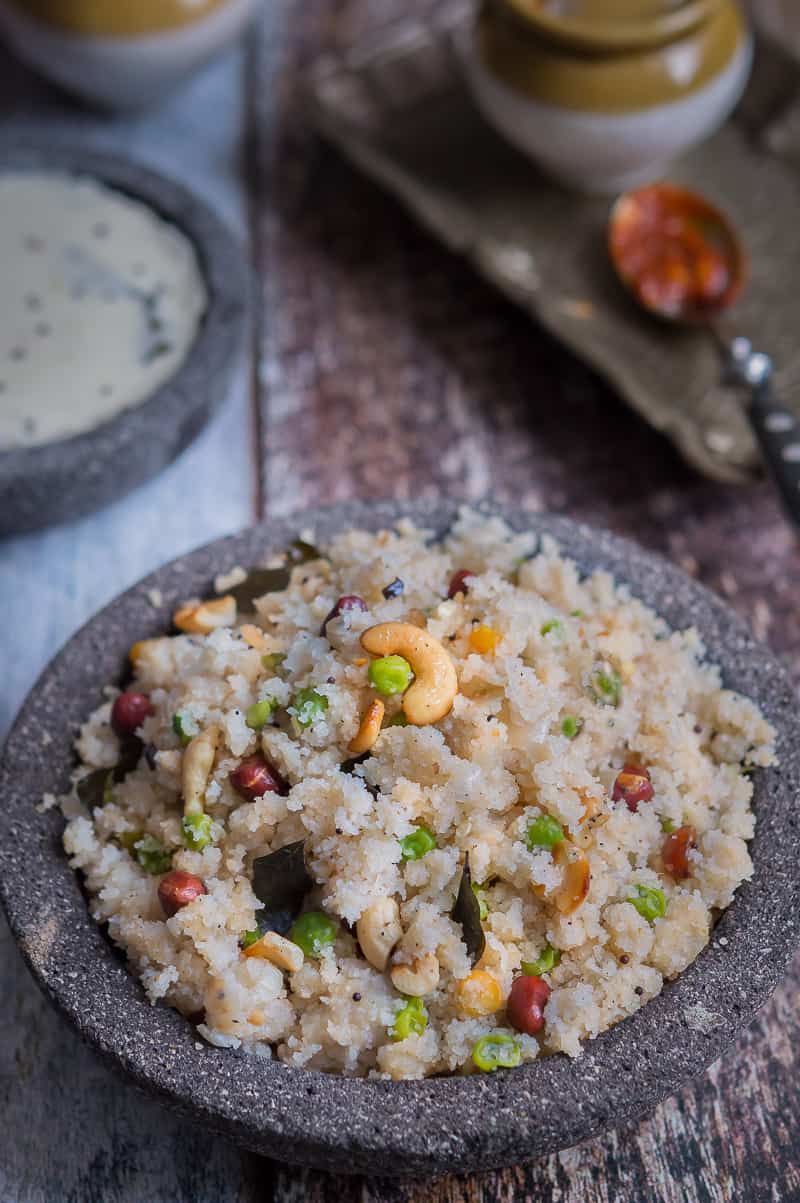This high-definition image, likely taken by a food blogger, depicts a meticulously presented grain dish, resembling porridge but with more texture, in a striking dark black stone bowl. The dish features a light beige-tan color and is lavishly garnished with green peas, red kidney beans, and cashew nuts, possibly hinting at a hearty combination of grains like polenta, grits, or sticky rice. The setting exudes an elegant rustic charm, with the bowl placed atop a dark brown wooden table made of raw planks, and surrounded by a softly blurred background created by a bokeh effect. The background reveals additional white bowls with intricate brown leaf designs, trays, jars of spices, and a spoon with a sauce or spice on it. A spoon is subtly present in the backdrop, enhancing the overall gourmet appeal of the scene.